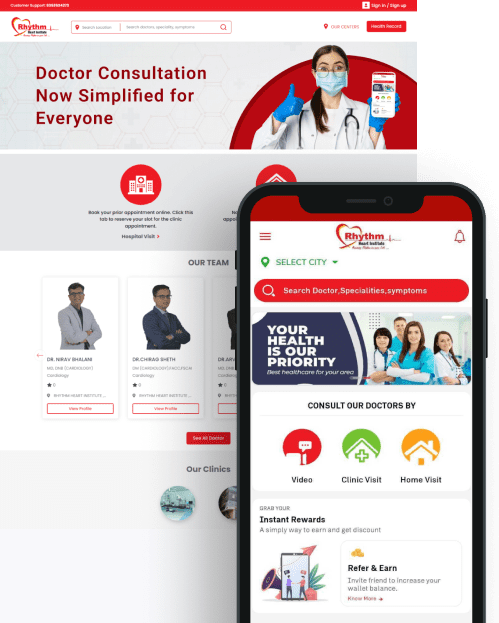The image features a vibrant layout for a medical consultation webpage. At the top, there is a red header followed by a white section displaying the word "rhythm." Adjacent to this is a search bar. Below this header, the background shifts to gray with prominent red text reading, "Doctor Consultation now simplified for everyone." 

Centered in the image is a female doctor, clad in a white lab coat with a stethoscope around her neck. She is also wearing a surgical mask and gloves, holding a smartphone up towards the camera in one hand, while giving a thumbs-up with the other hand. 

In front of her, prominently displayed, is a black smartphone screen showing the same webpage. This screen mirrors the layout with a red header, white background, and a red search bar. Beneath the search bar, there is an image of healthcare professionals in scrubs, accompanied by the text, "Your health is our priority." Below this image, additional information is provided: "Consult our doctors by video, clinic visit, home visit," and it highlights benefits like "instant rewards" and "refer and earn.”

The overall presentation emphasizes the ease and accessibility of modern medical consultations through various formats, and showcases a professional, user-friendly interface.